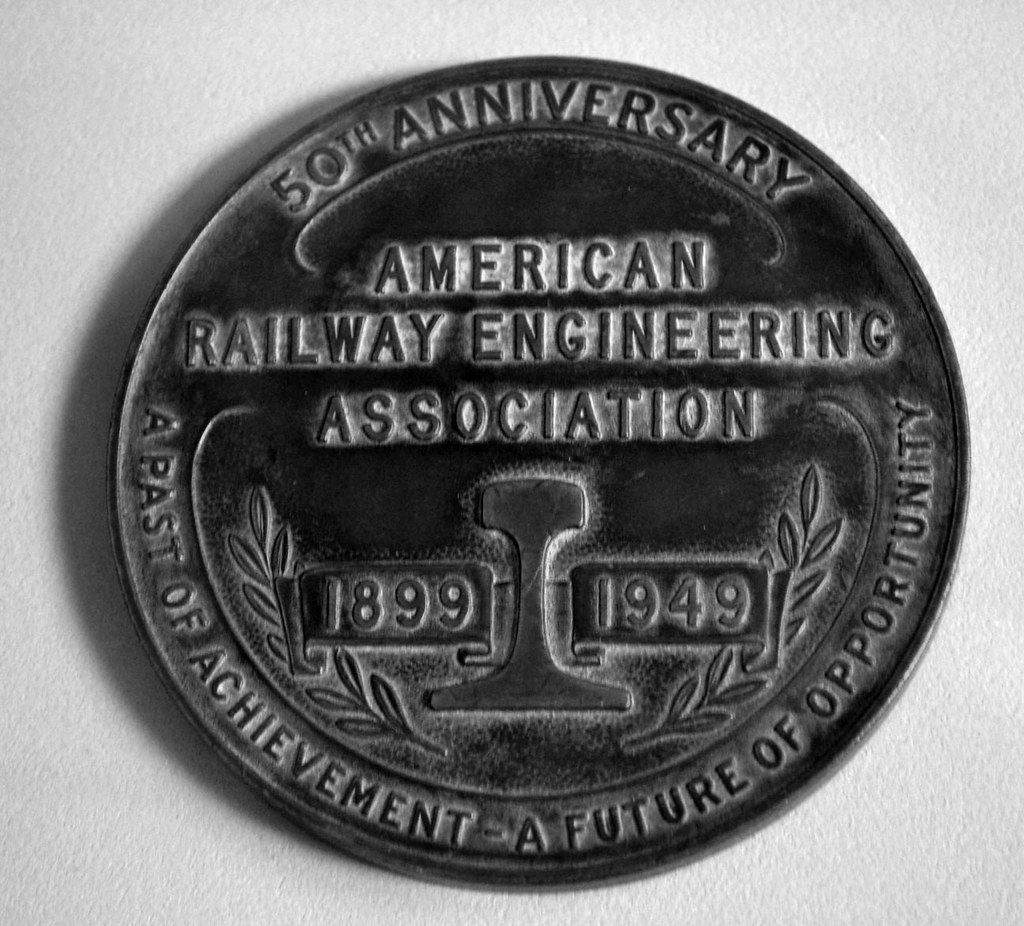The image depicts a close-up of a commemorative circular metal plaque in an older dark metal color, displayed against a white plaster wall background. The plaque features raised lettering and intricate design details. At the top, it reads "50th Anniversary." Beneath this, centrally aligned, is "American Railway Engineering Association." Below this text, there is an emblem resembling an anvil paired with a scroll, often mistaken for a railroad tie or a chess piece. The scroll flanks the anvil with the years "1899" on the left and "1949" on the right. Along the curve at the bottom of the plaque, the motto "A Past of Achievement, A Future of Opportunity" is inscribed, emphasizing the association's historic milestones and forward-looking vision. Overall, the plaque appears solemn and enduring, draped in elements that highlight the significance of the occasion it commemorates.